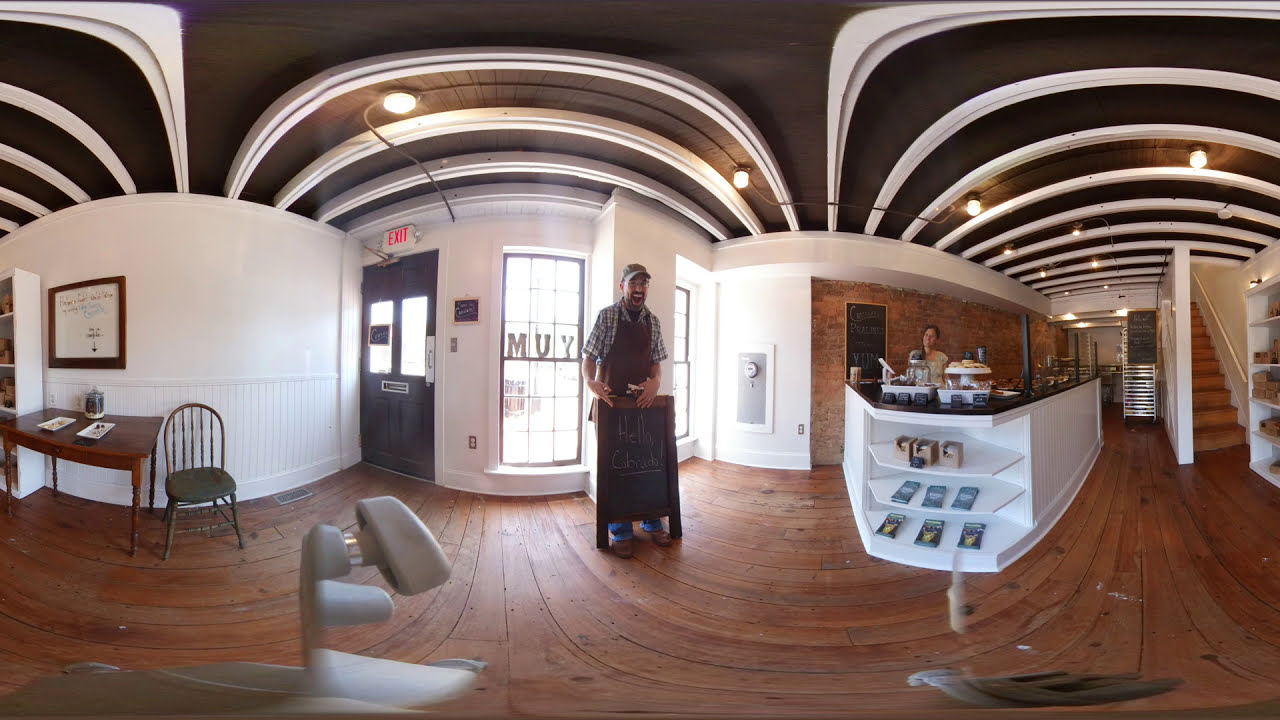This detailed photograph captures the elegant and modern interior of a cafe or bakery that is divided into three segments. At the center, a doorway with a large display window showcases the letters M-U-Y, flanked by dramatic arched ceilings with recessed lighting. Immediately inside the entrance stands a man with a beard, wearing a short-sleeve checked shirt, apron, baseball cap, and spectacles. He is smiling and pointing at a blackboard on an easel with the partially readable message "Hello CUPRA." The floor, composed of polished wooden planks, complements the room’s sophisticated aesthetic.

To the left, adjacent to the entrance, is a white wall adorned with framed certificates and a painting. Against this wall, a cushioned chair and a wooden desk sit, complete with trays and a container. A bookcase partially visible from the camera’s angle adds to the decor.

The right segment of the room features a U-shaped reception counter with a brown top and white sides, mirroring the color scheme of the walls and arches. The counter displays an array of desserts, confectionaries, and bookshelves stocked with various reading materials. A woman stands behind it, framed by the white partition wall housing a staircase to an upper floor. Behind her, there are industrial stainless steel appliances indicating that this establishment is likely a bakery or a coffee shop. The daylight streaming through the windows, combined with the ample recessed lighting in the black-and-white designed ceiling, illuminates the entire space, emphasizing its warm, inviting atmosphere.